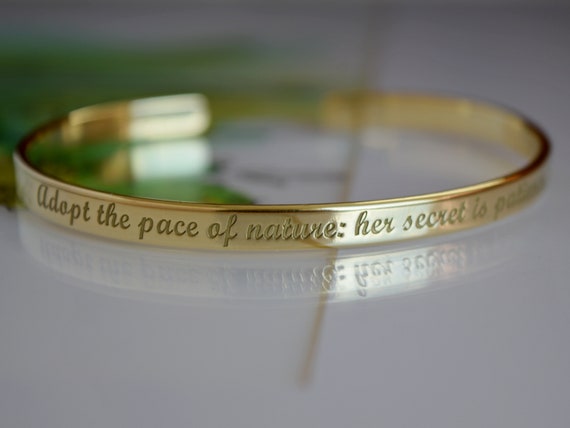The photograph showcases a delicate, thin gold bracelet resting on a reflective glass surface with an underlying white background. The bracelet, which lacks a clasp and is meant to be slid over the wrist, features an inscription in elegant cursive that reads, "adopt the pace of nature: her secret is patience." Only the front part of the bracelet is in sharp focus while the text at the back becomes blurry, creating a slightly challenging read. The engraved words are meticulously detailed. Surrounding the bracelet, and blurred in the background, are indistinct green leaves or foliage and possibly a small brown twig, adding a naturalistic element to the image. This serene and reflective composition emphasizes the theme of patience and harmony with nature.